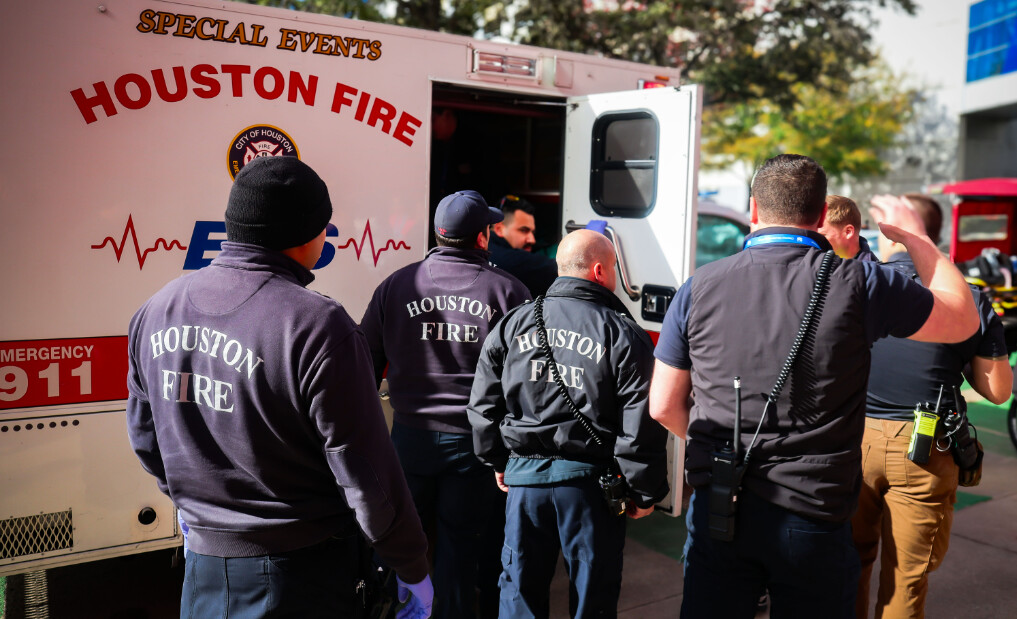The image depicts a vibrant outdoor scene featuring the Houston Fire Department at a community event. Central to the image is a white ambulance adorned with the phrases "Houston Fire Special Events" in red and "EMS" in blue, along with a red heartbeat line and "Emergency 911." Surrounding the vehicle are six individuals, some donning jackets and hoodies with "Houston Fire" emblazoned on the back in capital letters. They are dressed in navy blue pants while one person sports a dark-colored cap and another wears a khaki coat. Various tones of blue, red, black, and green are prominently featured in the attire and elements of the scene. The backdrop showcases leafy green trees and a concrete sidewalk, bathed in daylight, adding to the overall sense of an organized and dynamic public safety demonstration.